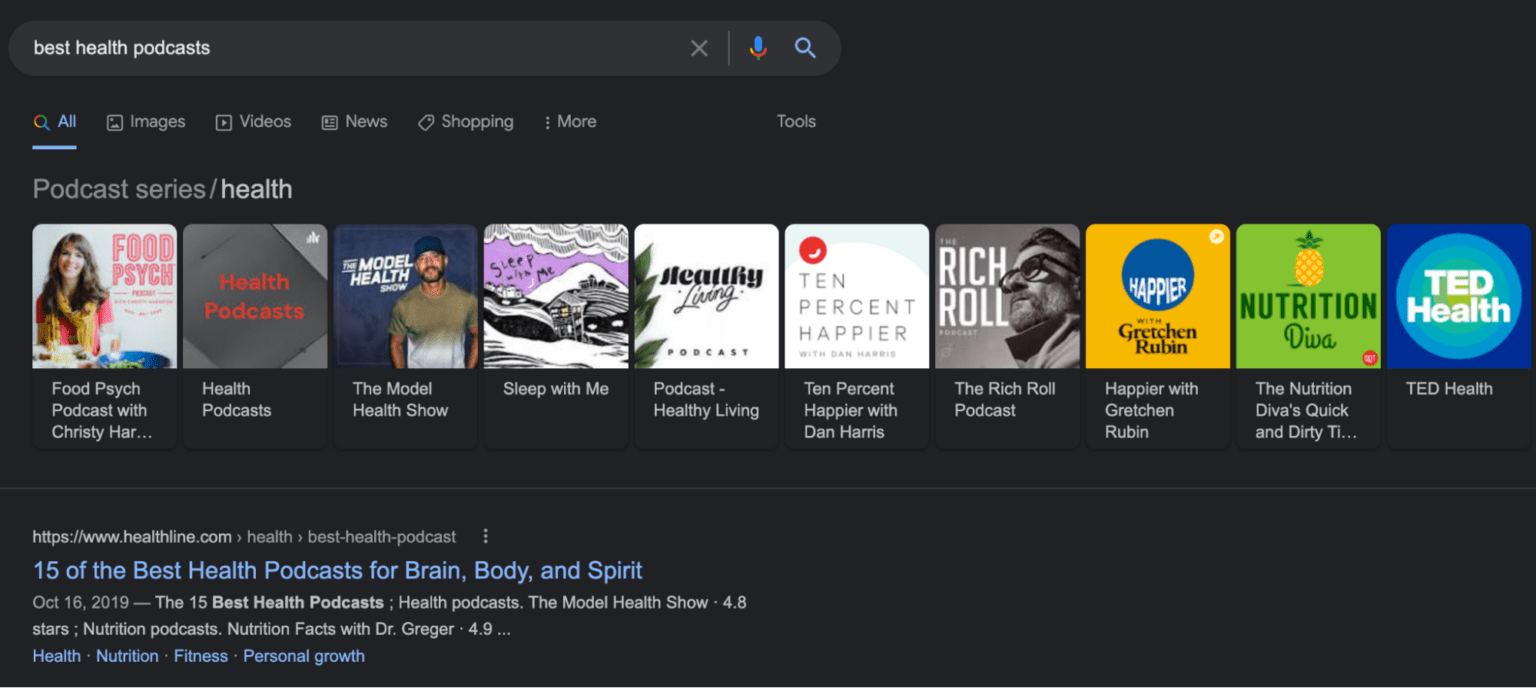In this screenshot, we observe a rectangular black image displaying a search results page with gray and blue text. In the upper left corner, there's a search bar with white text on a black background containing the query "Best Health Podcasts". Directly below this is highlighted blue text labeled "All". To the right of this blue text, various options appear in gray text: "Images," "Videos," "News," "Shopping," "More," and "Tools".

Below this set of tabs, larger gray text reads "Podcast Series / Health", indicating the category of the search results. The search results for health podcasts are presented in a horizontal list, featuring the following podcasts from left to right:

1. "Food Psych Podcasts with Christy Harrison"
2. "Health Podcast"
3. "The Model Health Show"
4. "Sleep With Me"
5. "Healthy Living Podcast"
6. "10% Happier with Dan Harris"
7. "The Rich Roll Podcast"
8. "Happier with Gretchen Rubin"
9. "The Nutrition Diva's Quick and Dirty Tips"
10. "TED Health"

This detailed layout provides a comprehensive view of the related health podcast options available based on the search query.